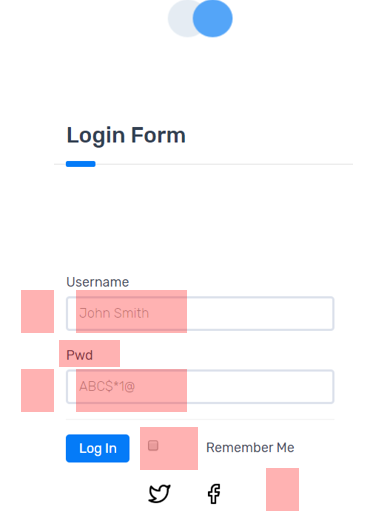The screenshot snippet displays a section of a white-background webpage, likely a login form, though the website itself is unidentified as there are no headers visible. At the top center, two overlapping circles are presented, with the left circle in a very light gray hue and the right in turquoise blue. Below these circles, "Login Form" is written in medium gray font. 

Underneath the title, a thin, very light gray horizontal line stretches from left to right, with a small segment on the right colored blue. Beneath this line, the login form comprises two outlined gray rectangles with solid light pink overlays on the left side. The top rectangle is labeled "Username," and the bottom rectangle is marked "PWD." Below the rectangles, there is a turquoise blue rectangular button with white font that says "Login."

On the right side of the form, "Remember me" is written in very light gray font. Below this, two outlined icons feature—the Twitter logo and the Facebook logo, represented by the letter "F."